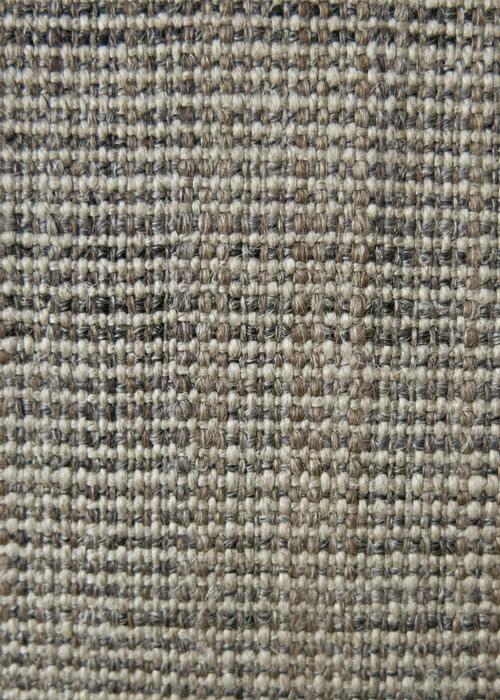This vertical rectangular image is a close-up photograph of a woven fabric, specifically a nubby upholstery or tweed-like material. The fabric's orientation is portrait, filling the entire frame with no additional objects or lettering. The woven texture exhibits a detailed interplay of colors: horizontal lines alternating between white and grayish-brown, interspersed with vertical beige threads. These beige threads contribute to an overall light beige appearance. Additionally, darker threads, ranging from dark gray to near black, interlace with the primary colors, adding depth and dimension to the fabric. The material appears robust and sturdy, potentially suitable for various uses such as indoor or outdoor carpets, seat covers for vehicles, or even as part of a man's jacket or upholstery for furniture. The photograph, characterized by representational realism, captures the intricate details and earth tones of the fabric, evoking a versatile and timeless aesthetic.